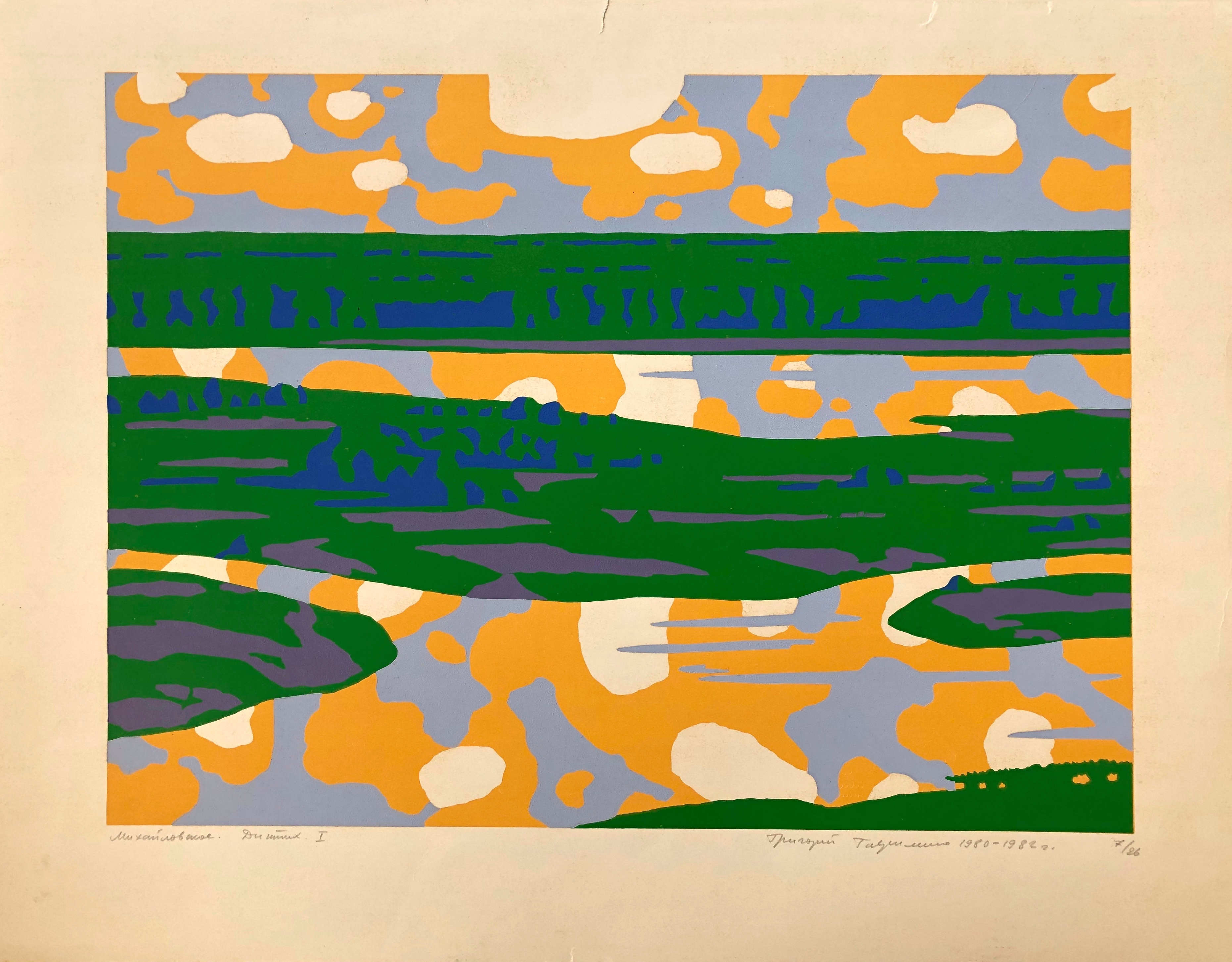The rectangular painting, set in a light tan frame, is a compelling piece of abstract art. The background is a complex interplay of various colors: grayish-blue and orange form the base layer, with random splotches scattered across, evoking the appearance of bodies of water dotted with little islands. Over these, circular splotches of beige and streaks of bright green—reminiscent of summer grass—add texture and dimension. The green is interwoven with gray streaks, resembling sand traps, and is further embellished with blue striations and shapes, which vary from linear patterns to round puddle-like areas. Additional purple shapes mingle within these bands of green. The layout includes several horizontal green bands, with one a quarter of the way down from the top, stretching across the entire width, while others only partially span the image, contributing to the dynamic, layered composition. The artist's signature is located at the bottom, although it is too small to be legible.